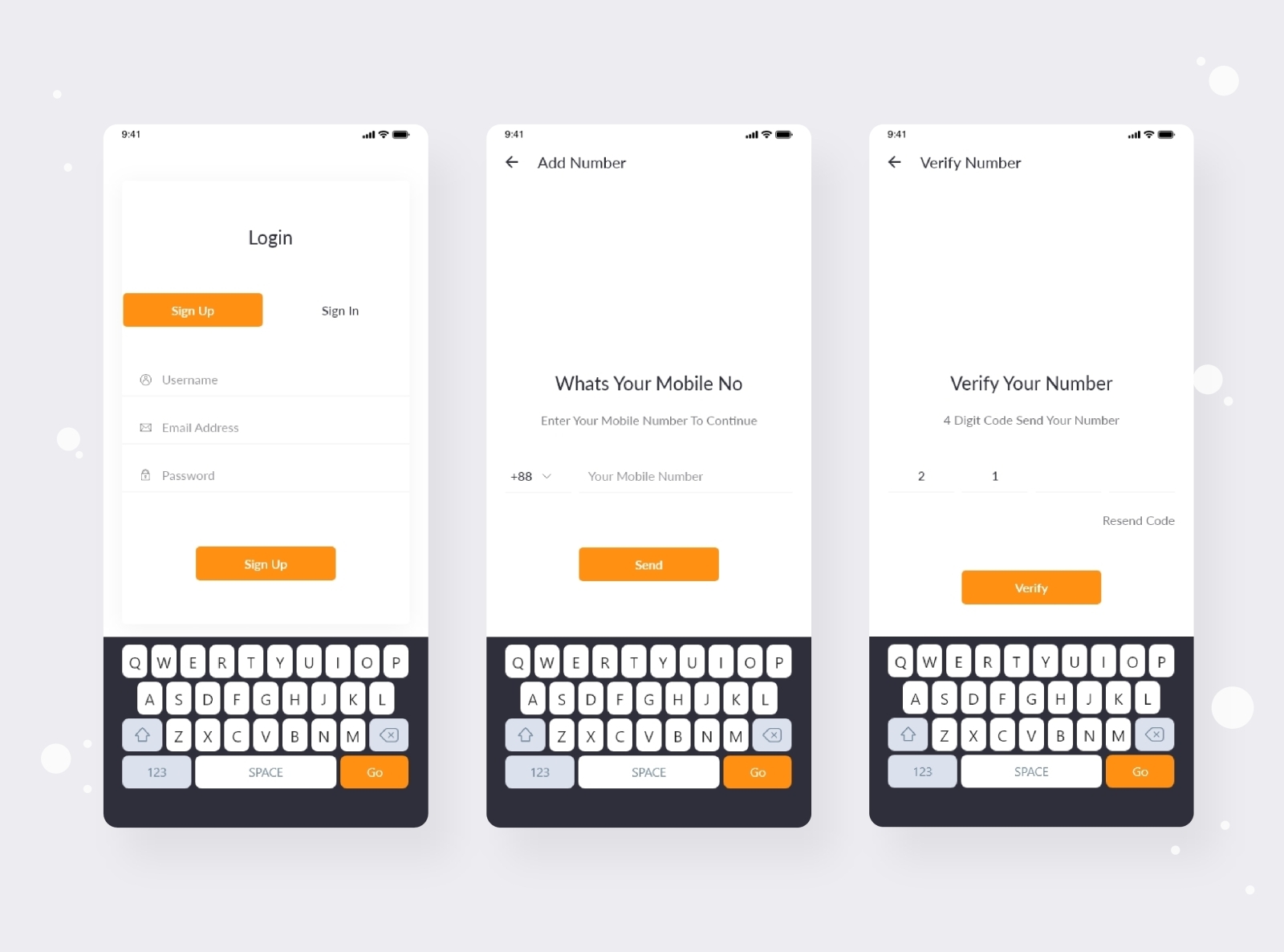The image features three mobile phones displayed against a gray background adorned with white bubbles. Each phone screen depicts a different step in the account login and verification process.

The first phone screen shows the initial login interface where users are prompted to enter their username or email address and password, followed by a sign-in button. A virtual keyboard is visible at the bottom for input.

The second phone screen asks users to input their mobile number. There is a designated field for entering the number, with options to either send or save the information once entered.

The third phone screen is dedicated to number verification. It instructs users to enter a four-digit code sent to their mobile number into an on-screen field, followed by a verify button.

The image collectively illustrates a simplified, generic login and verification sequence across the three mobile phones.